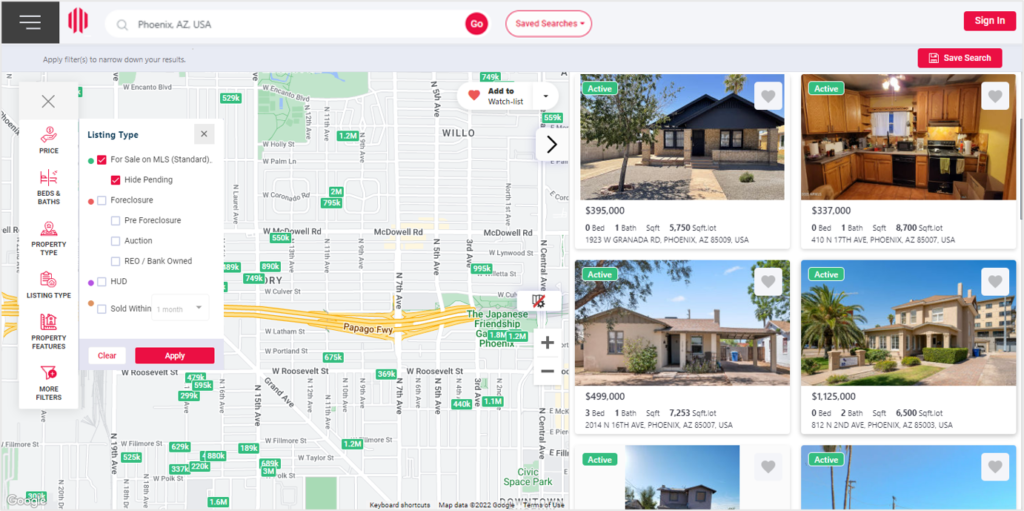The image depicts a detailed view of a real estate web page interface. At the top, a small gray square featuring three horizontal bars serves as a menu icon. To its right, a search bar is prominently displayed, accompanied by a circular red logo. The search bar currently indicates a query for properties in Phoenix, Arizona, USA. Next to the search bar, a red "Saved Searches" dropdown button is visible, followed by a red "Sign In" button.

Below these elements lies an interactive map highlighting different neighborhoods within Phoenix. The map is overlaid with several red icons representing various real estate filters such as price, bed and bath, property type, listing type, property features, and more.

The "Listing Type" filter is expanded, revealing options like "For Sale" and "High Pending," both of which are selected. Additional options include "Foreclosure," "Pre-Foreclosure Auctions," "Bank-Owned," "HUD Housing," and "Sold When." At the bottom of the filter menu, a red "Apply" button allows users to set their chosen filters, while a white "Clear" button offers the option to reset all selections.

On the right side of the page, several property listings are visible. Among them, one property is listed for $395,000 and another for $337,000. The overall interface is clean and organized, designed to assist users in efficiently searching for properties in the Phoenix area.